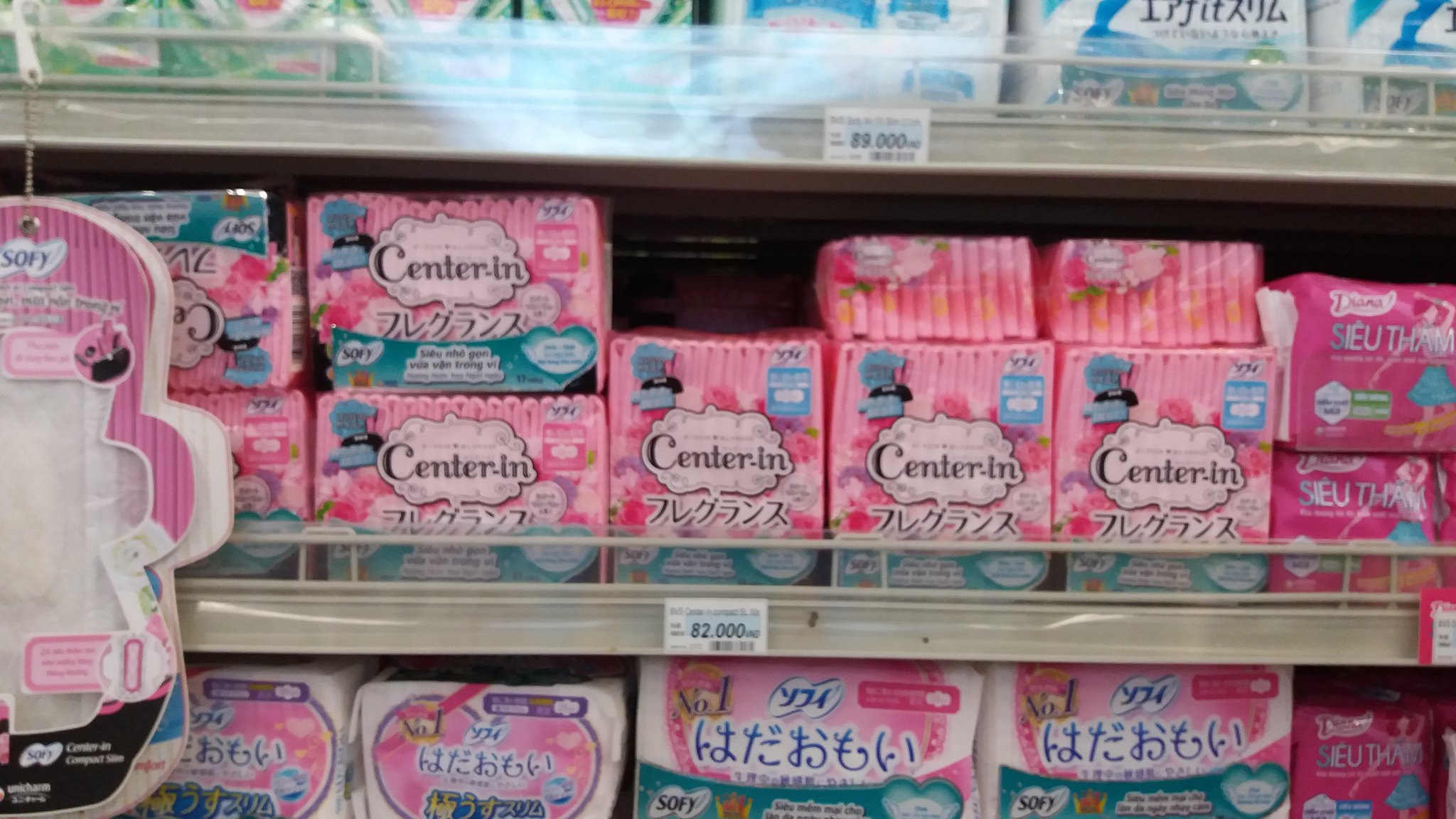The image captures three shelves in a supermarket, displaying a variety of packaged products, predominantly diapers. The central focus is a middle shelf filled with light pink packaged diapers from the brand "Center Inn." The packaging features a clear cellophane wrap revealing individually wrapped pink items inside, with a white cloud-like label stating "center-in" in black letters. Prices, marked as 82,000, suggest a non-European currency. The lower shelf contains larger, plastic-wrapped products decorated with pink circles and green text. The top shelf has similarly stacked items in blue and green packaging, marked with prices such as 89,000. The shelves themselves are made of white metal with a lip design to prevent items from falling. Hanging from the shelf above is an additional pink item marked "softy," suspended by a silver thread.